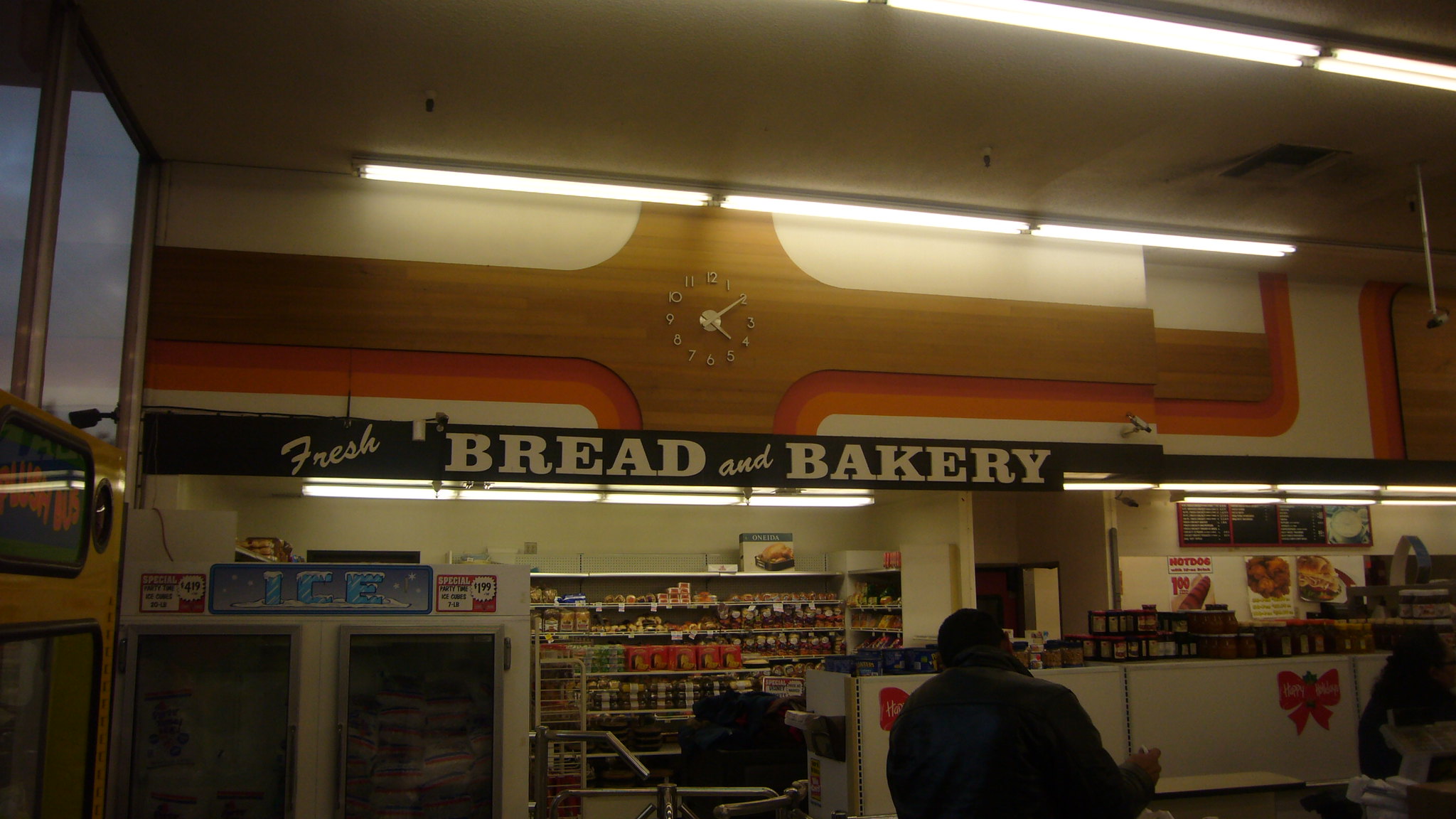This vintage-style photograph captures the interior of a grocery store, characterized by its dim, warm lighting that casts yellowish-green hues throughout the space. The decor features large, curvy stripes in retro red and orange tones reminiscent of the 1970s, adding a touch of nostalgic charm to the setting. Prominently displayed on the wall is a sign reading "Fresh Bread and Bakery," indicating the section of the store. Above this sign, a large wooden clock shows the time as approximately 4:10. In the bottom right corner of the image, a few tables are visible, with a glimpse of customers seated and engaged in quiet conversation.